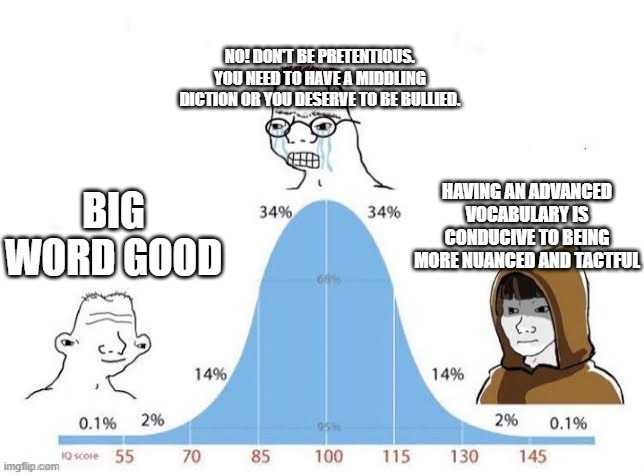The image displays a blue graph that explores the relationship between articulation and the use of large words, specifically questioning whether employing an extensive vocabulary enhances communication or simply results in pretentiousness. The graph spans IQ scores from 55 to 145, with increments marked at 15-point intervals. The numbers on the graph are presented in brown.

At the graph’s midpoint, representing an average IQ score of 100, a cartoon character with exposed teeth and glasses is featured. This character is accompanied by a bold, white text on a black background stating, "NO, DON'T BE PRETENTIOUS. YOU NEED TO HAVE A MIDDLING DICTION OR YOU DESERVE TO BE BULLIED." 

The graph illustrates statistical data indicating that 34% of individuals are positioned on each side of this midpoint, 14% further away, 2% more distant, and just 0.1% at the extremes.

On the left side of the graph, there is a caricature of a person with a disproportionately high forehead, wide-set eyes, and an exaggerated nose, suggestive of a Neanderthal. Above this drawing, in larger type, it reads, “BIG WORD GOOD,” implying that individuals with lower IQ scores might simplistically regard large words as superior.

Conversely, on the right side, a character resembling a girl in a brown hood asserts, "HAVING AN ADVANCED VOCABULARY IS CONDUCIVE TO BEING MORE NUANCED AND TACTFUL," suggesting that individuals with higher IQ scores may appreciate the value of an extensive vocabulary.

Overall, the graph aims to provoke thought on whether the use of sophisticated language serves to improve articulation or merely acts as a veiled attempt at appearing more intelligent, potentially leading to derision.